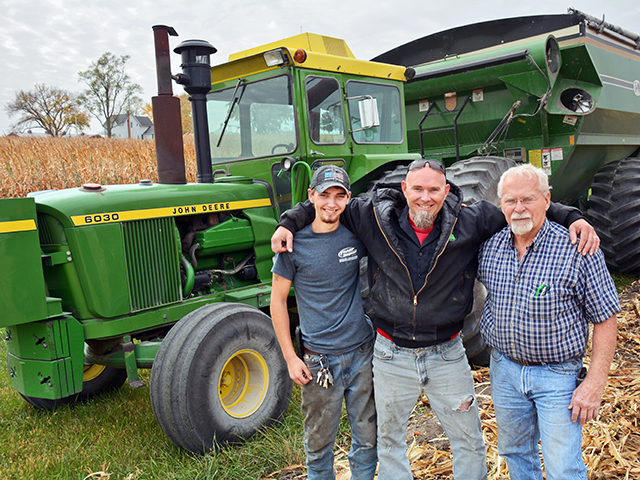This photorealistic image captures three Caucasian men standing on a farm in front of a large green John Deere tractor, which features yellow detailing and a prominent smokestack. The tractor is pulling a large green agricultural container with a red and black stripe at the top. Behind the machinery, a field of grains or hay is visible, along with a scattering of trees and some distant farm buildings under a cloudy sky.

The men appear to be related, suggested by their close physical proximity and mirrored poses. On the right stands an older gentleman, likely in his late 60s or early 70s, with white hair, a white goatee, and glasses. He is dressed in a blue and light blue striped collared shirt, left unbuttoned at the top, and blue jeans. His left arm rests by his side.

In the middle is presumably his son, in his 40s, bald and sporting a black and white goatee. He is wearing a black jacket over a shirt with sequined blue and red accents, and ripped light blue jeans. His glasses rest on top of his head. He has interlocked arms with the men on either side.

To the left is the youngest man, potentially in his early 20s, wearing a blue t-shirt, dirty blue jeans, and a black baseball cap. A keychain dangles from one of his pockets. The three men are standing on a subtle mix of cornstalks and grass, with the vast expanse of the farm stretching out behind them.